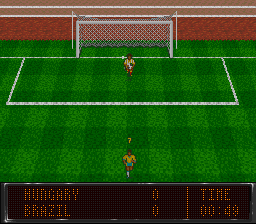The image depicts an arcade-style soccer game featuring a virtual match between Hungary and Brazil. The scene shows only two players, one positioned as a goalie and the other situated at the bottom of the screen, both donned in bright yellow uniforms. The player at the bottom has a question mark icon above their head, suggesting a moment of confusion or decision-making in the game. The scoreboard at the bottom indicates a tied score of Hungary 0, Brazil 0, with an in-game time display showing 48 seconds elapsed. The playing field appears vividly green, typical of digital soccer games, and a brick wall can be seen in the background, reinforcing the arcade aesthetic. This game's simplistic yet nostalgic design evokes classic soccer games found in arcades.